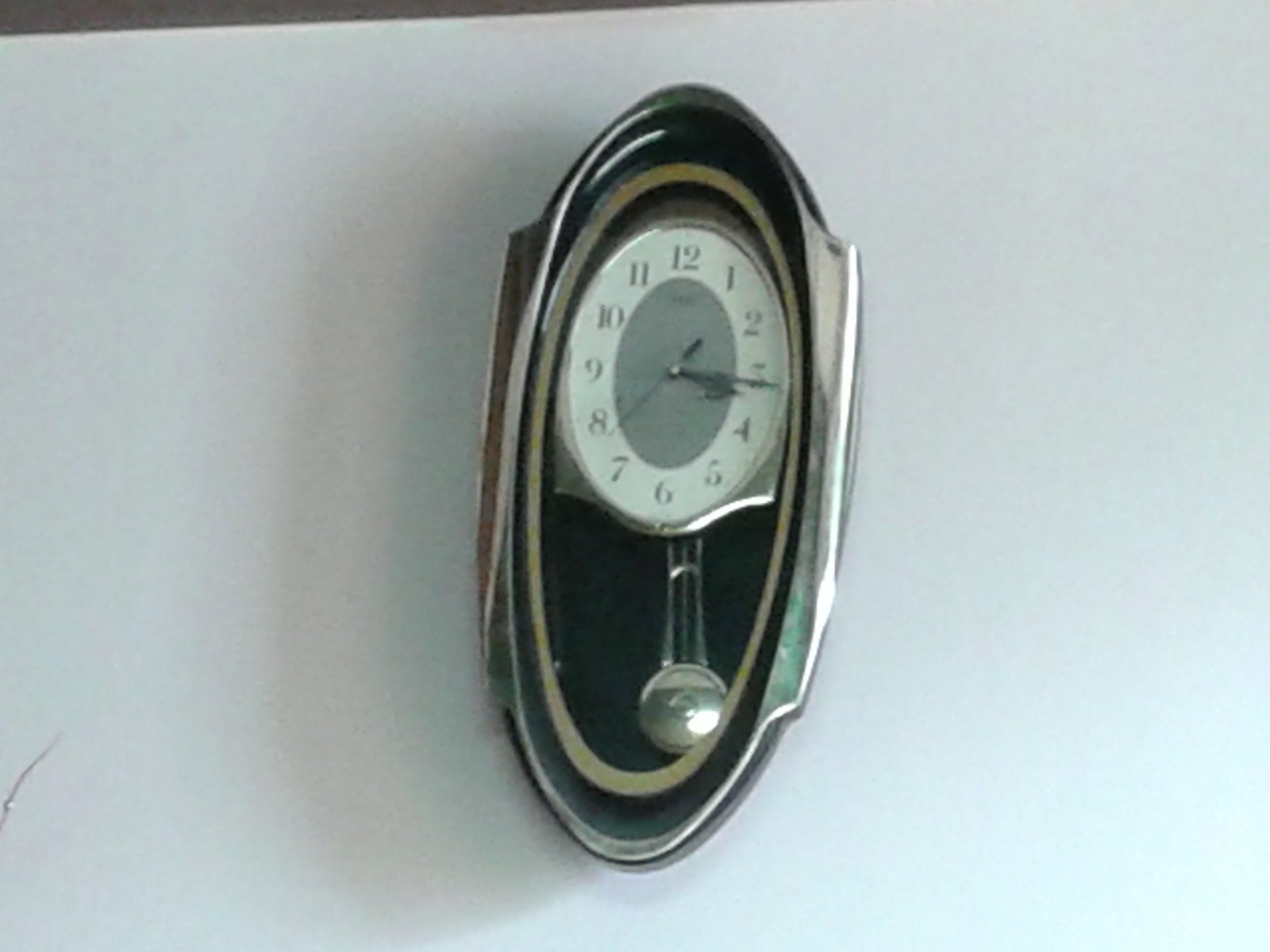The image showcases a vintage wall clock mounted on a smooth, white plaster wall that occupies most of the frame. The clock, prominently positioned in the center, features a vertically oriented oval shape with a textured silver and black border, suggesting an aged or tarnished appearance with hints of gold. The clock face, also oval in shape, has a white background with large black numbers in a classic font, reading 3:15, though the minute hand is closer to the 8, indicating approximately 3:16. Central to the clock face is a gray oval, adding depth to its design. Dangling from the bottom of the clock face is a silver pendulum, slightly swung to the right, housed within a black backdrop inside the clock's case. Notably, the bottom left corner of the white wall displays a small crack, hinting at the passage of time. The overall scene is well-lit but captured in a low-quality image, adding to the clock's nostalgic charm.